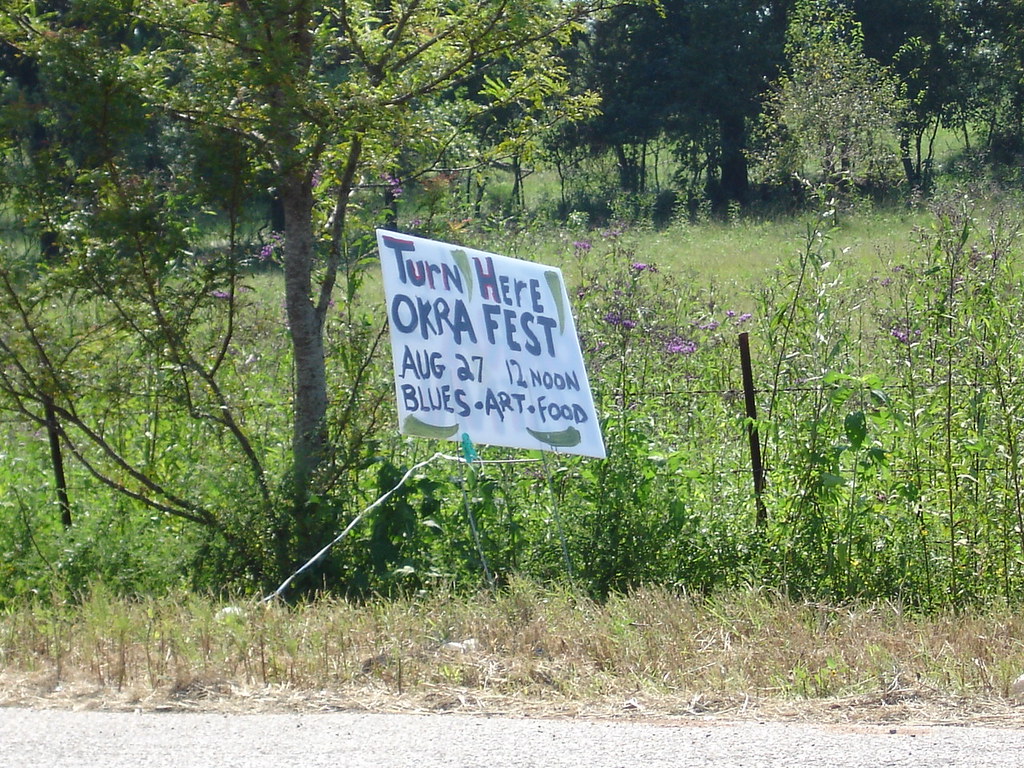A horizontal image captured in the countryside along a gravel road. In the foreground, a barbed wire fence runs across the lower center of the image, with lush green weeds and shrubs thriving at its base. A single, robust tree stands slightly left of center, accentuating the verdant surroundings. Behind the barbed wire fence, various green weeds and grasses flourish, leading up to a distant tree line and an additional fence. Centrally positioned and tied to this second fence or a post, a large white sign tilts backwards at an angle. The sign features curved, pizza-shaped green objects, which are identified as okra. Bold black letters on the white sign instruct readers to "Turn Here, Okra Fest." Below this directive, additional details are provided, highlighting the event's date, "August 27th," and time, "12 Noon," as well as the festivities which include "Blues, Art, and Food."